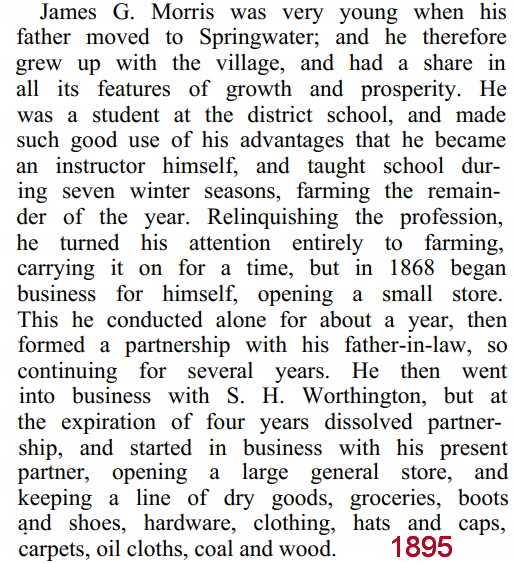The image is a black-and-white, single-column, justified newspaper article printed in an 8-point font on a white, borderless background. At the bottom right corner, it features a red stamp with the year "1895". The article recounts the life of James G. Morris, detailing how he grew up in the village of Springwater after moving there with his father. Morris attended the district school, where he excelled to the point of becoming an instructor, teaching during seven winter seasons while farming the rest of the year. Shifting his focus entirely to farming, he later opened a small store in 1868, which he ran alone for about a year before partnering with his father-in-law for several years. Subsequently, he entered into a business venture with S.H. Worthington, which lasted four years. After dissolving that partnership, Morris started a new business with his current partner, establishing a large general store that offered an extensive range of products, including dry goods, groceries, boots and shoes, hardware, clothing, hats and caps, carpets, and oilcloths.